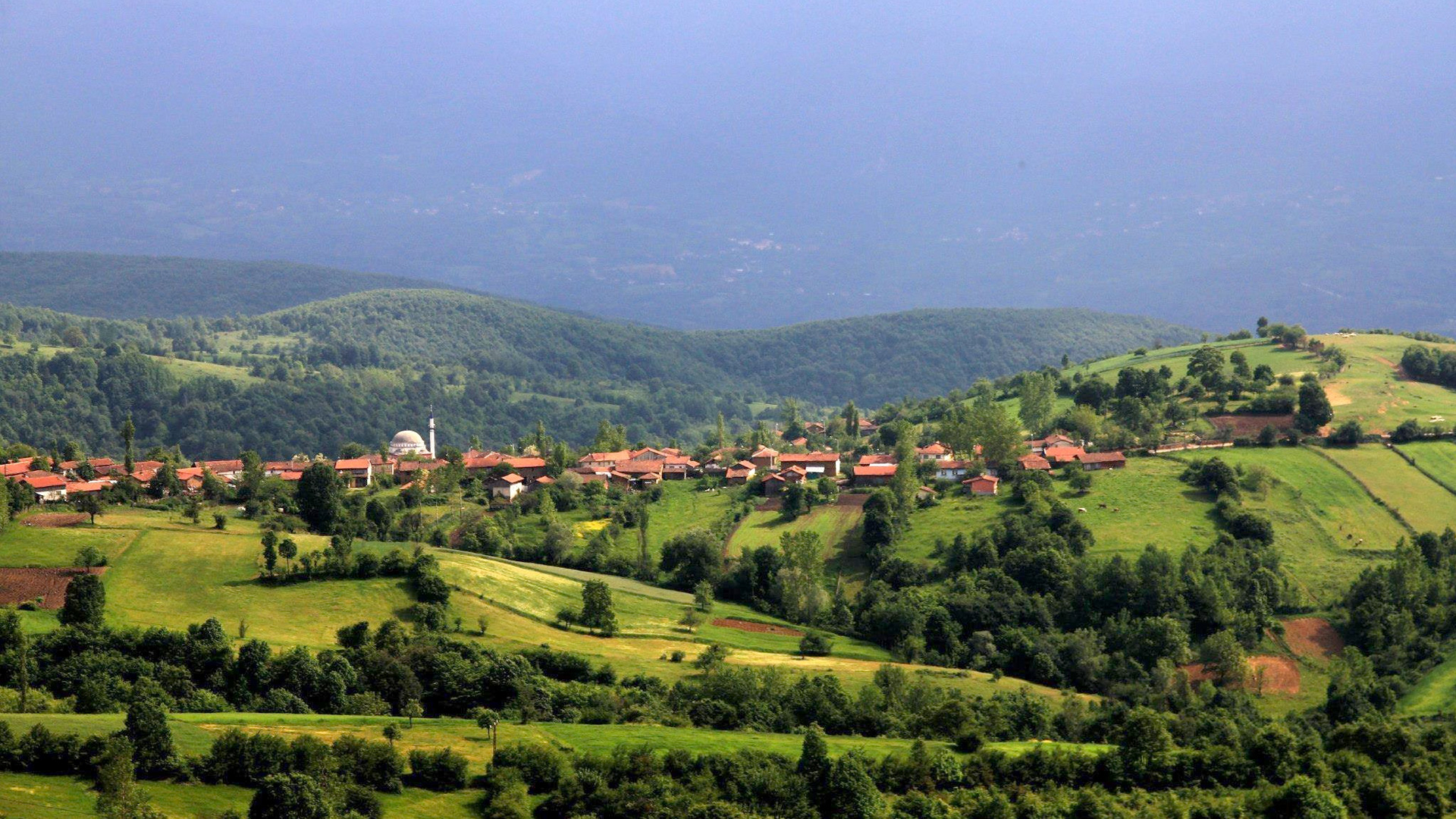The image depicts a serene landscape featuring rolling green hills adorned with lush, dark green trees and light green grass. Scattered across the hills are numerous houses with distinctly red, triangular roofs. One notable structure towards the left side of the image is a white building with a dome-shaped roof and an adjacent pole, resembling a church. The foreground of the image showcases various patches of grass and trees, including some areas where the grass appears shorter or absent, marked in a square pattern and displaying different shades of green and brown. In the background, additional hills stretch into the distance, becoming increasingly hazy and foggy, suggesting the presence of very distant cities. Small pathways wind through the landscape, adding to the picturesque quality of the scene.